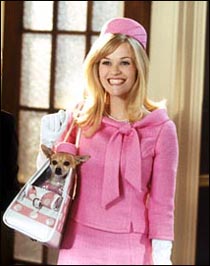This image captures Reese Witherspoon as Elle Woods from the movie Legally Blonde. She is donning a stylish, long-sleeved pink two-piece skirt suit paired with a matching pink tie around her neck. Complementing her ensemble is a small pink pillbox hat perched on her head. Her blonde hair, parted on the side, cascades down to her collarbone. Her radiant smile reveals her teeth. Elle accessorizes with elegant white elbow-length gloves and a pearly necklace. She holds a pink-and-white striped handbag, inside which sits her chihuahua, dressed similarly in a matching pink hat. Behind her is a framed door adorned with glass panes and a white lace curtain.